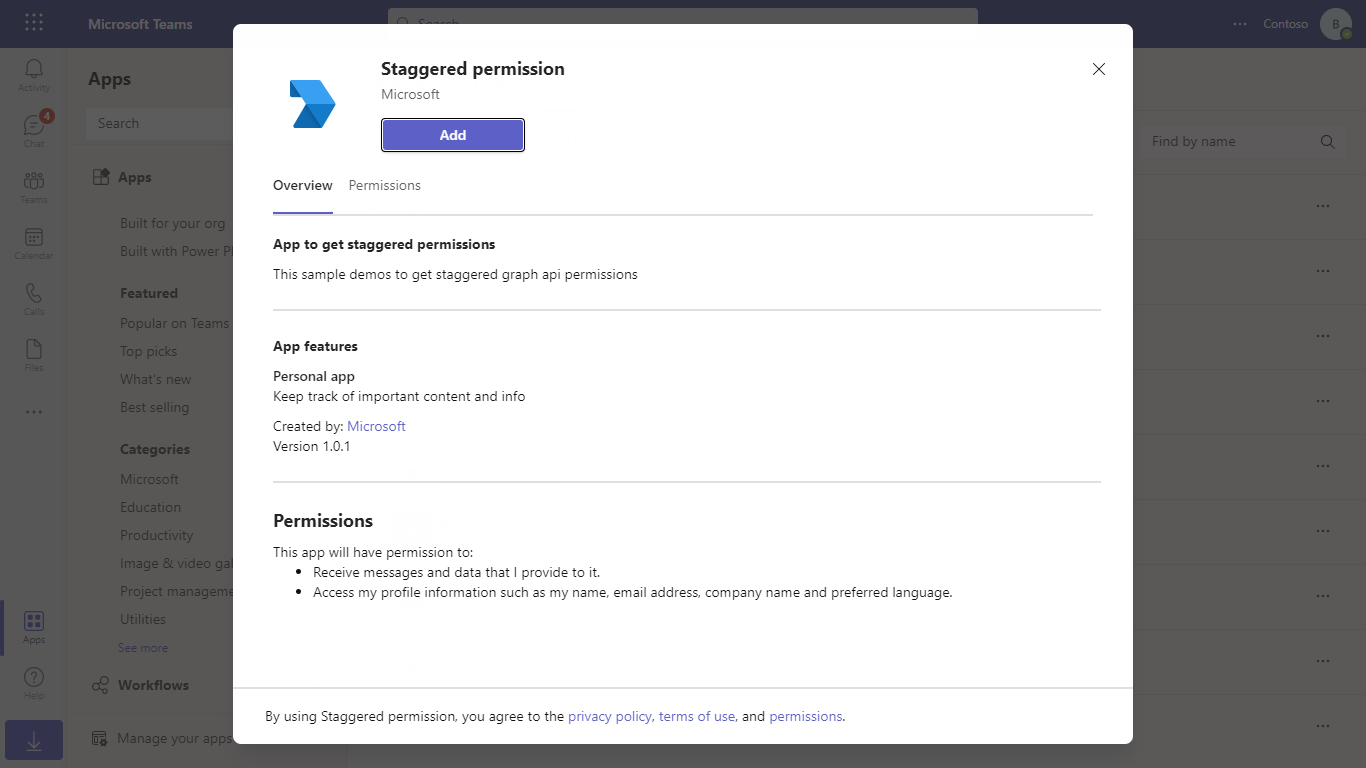The image depicts a pop-up window on a Microsoft Teams interface, focusing on the "Staggered Permissions" app. The pop-up features a white box with detailed information. At the top, it prominently displays a blue geometric logo on the left, followed by the text "Microsoft" and a purple "Add" button. The pop-up has two tabs: "Overview" and "Permissions," with the "Overview" tab highlighted.

Under the "Overview" tab, it lists the app name "Staggered Permissions" and describes it as a sample demo to obtain staggered Graph API permissions. It also mentions that the personal app is designed to help keep track of important content and information. The app is created by Microsoft and is currently at version 1.0.1.

The permissions section specifies that the app will have access to receive messages and data provided by the user, as well as profile information such as name, email address, company name, and preferred language. Users are informed that by using "Staggered Permissions," they agree to the privacy policy, terms of use, and permissions.

In the background, the partially visible Microsoft Teams interface has a dark overlay. At the top, it shows "Microsoft Teams" and a search bar. In the upper right corner, "Contoso" is displayed. Below this, in a lighter area, there are sections for "Apps," with a search bar labeled "Apps" and options for "Build for your org" and "Build with PowerPoint." Additionally, there are sections for "Featured," "Categories," and "Workflow," along with various icons on the left side of the screen.